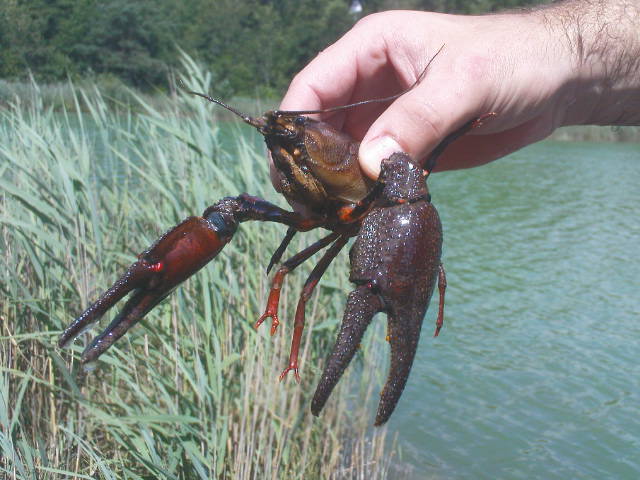A photograph captures a right hand, presumably male, holding a dark-colored lobster or crayfish between the thumb and forefinger. The hand, its arm adorned with visible hair, lifts the crustacean just above the surface of the water, suggesting it has been freshly retrieved. The lobster’s long antennae, claws, and several legs are clearly visible. To the left of the image, straw or seagrass contrasts with the bluish-green water on the right. In the distant background, a line of trees is discernible. The daylight is inferred from the reflection of the Sun, enriching the photograph with hues of brown, red, green, flesh tones, and the darker shades of hair.